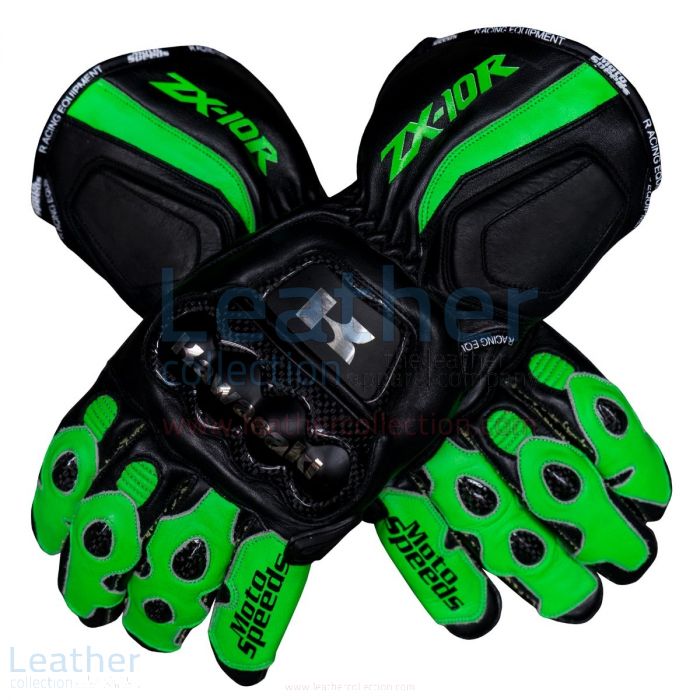The image showcases a pair of large, heavy-duty motorcycle gloves, predominantly black with striking lime green accents. The gloves are crossed over each other on a white background. The back of each hand features a prominent ‘K’ symbol surrounded by four black bubble designs. The fingers are mostly green with small black dots, and the pinky finger of each glove is emblazoned with the word "Motospeeds." Across the top near the wrist, the gloves display the text "ZX-10R" in green. The black leather sections of the gloves bear additional writing, including a watermark that says "Leather Collection," visible in the background and at the lower left corner of the image. These gloves are well-insulated, sturdy, and indicative of the ZX-10R leather glove collection, making them suitable for high-performance racing.